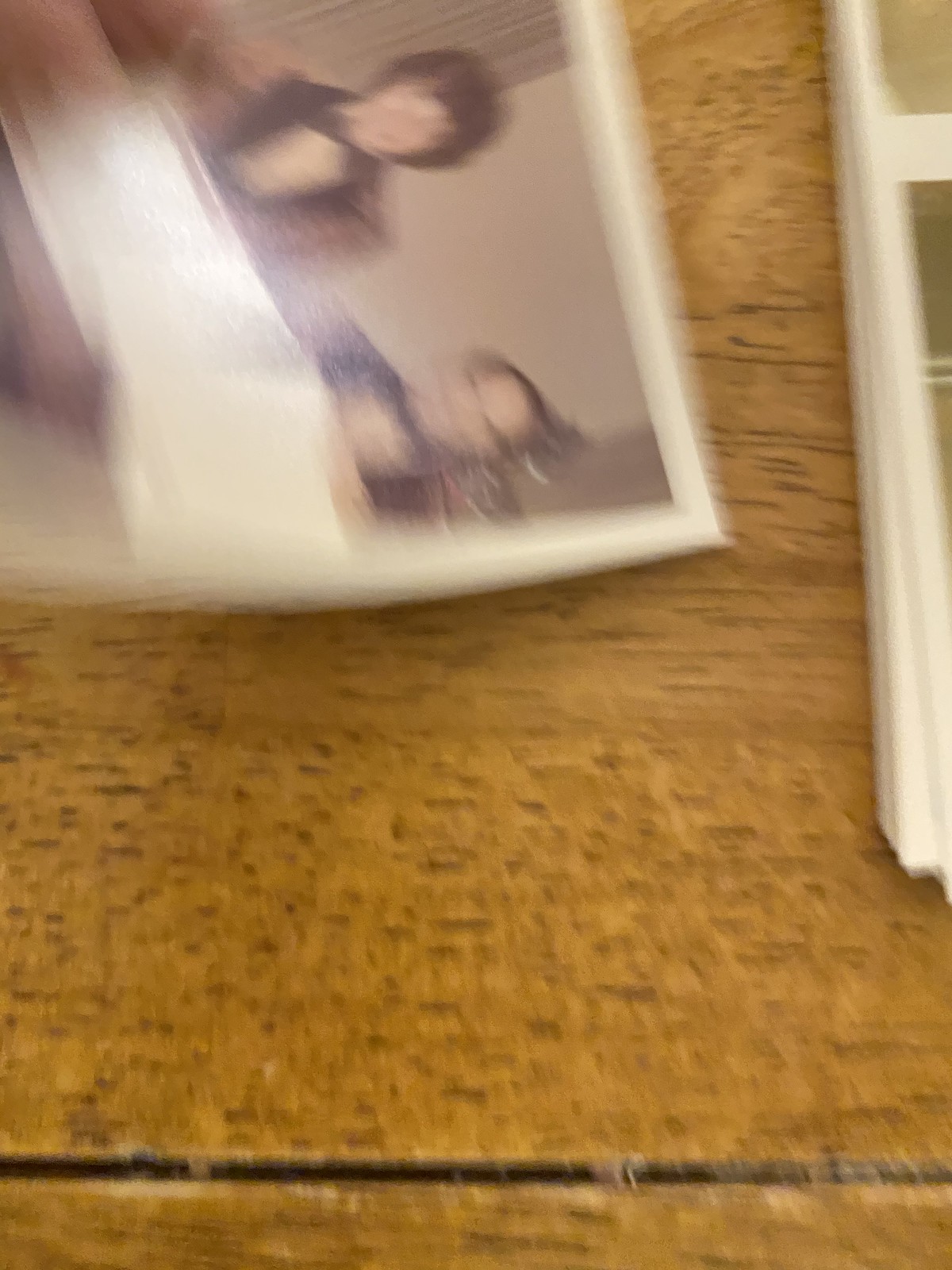This image captures an assortment of photographs resting on a wooden tabletop, with the wood grain running horizontally across the frame. At the very bottom of the image, a distinct black line marks the table's surface. The primary focus is a slightly crumpled Polaroid photograph positioned sideways, featuring a blurred man and woman smiling directly at the camera. This Polaroid photo is distinguished by its iconic white border. To the right of the main Polaroid, a small stack of similar white-bordered photos is visible, though only the edges of these additional photos are partially seen. The overall blurriness adds a nostalgic, dreamy quality to the scene.